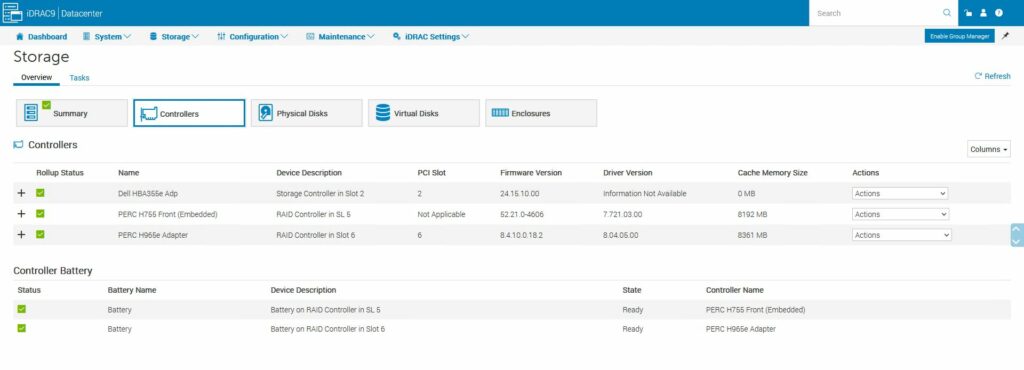The image displays a detailed screenshot of a program menu, primarily dominated by a blue bar at the top. In the upper left-hand corner of this blue bar, there's the name of a company that appears to be "ORAC9" followed by a word starting with "D". To the right of this, there's a white search bar. Further right, the blue bar features three icons: an unlocked white padlock, a white silhouette of a person, and a circular icon. Below the blue bar, the interface transitions to a gray section displaying a dashboard with multiple options such as System, Storage, Configuration, Maintenance, and iDRAC Settings. On the far right of this gray section, there's another blue icon that is hard to decipher and features a pen or similar icon next to it.

Beneath this area, there's a labeled section "Storage," with subcategories "Overview" and "Tasks." The "Overview" tab is currently selected. This section contains five gray boxes labeled from left to right: Summary (marked by a green box with a checkmark), Controllers (selected with a blue rim), Physical Disks (depicted with a disk icon), Virtual Disks (represented by a stack of four circles), and Enclosures (with an unclear icon). Below these categories, there's a detailed table for "Controllers" containing eight columns: Roll-Up Status, Name, Device Description, PCI Slot, Firmware Version, Driver Version, Cache Memory Size, and Actions. The row entries in this table appear with green check-marked boxes under the Roll-Up Status and additional details under each column. The "Actions" column features its own scrollable bar labeled "Actions."

Further below, there's another section labeled "Controller Battery," detailing another table with five columns: Status, Battery Name, Device Description, State, and Controller Name. Each row within this table includes green check-marked boxes under Status, with the Battery Name listed as "Battery" and State designated as "Ready."